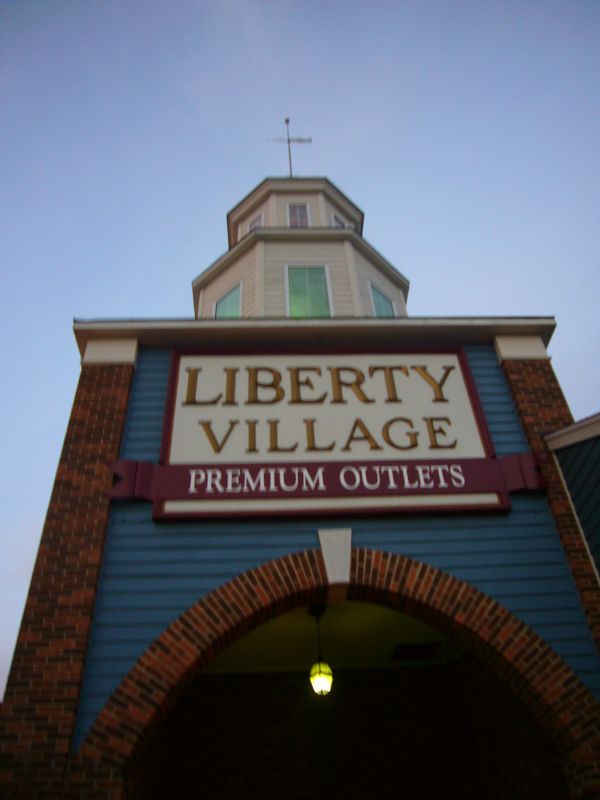The image depicts the facade of a building seen from a low vantage point, with a clear blue sky as the backdrop. The structure has a striking brick archway at the entrance, flanked by brick columns. Hanging from the arch is a lit ceiling light, illuminating a whitish ceiling within the darkened entrance. Between the brick columns, the building features blue siding adorned with a prominent white sign. The sign displays the text "Liberty Village" in gold or brownish lettering, followed by "Premium Outlets" in white. Above the sign and main structure, the roof ascends into two tiers, each hexagonal or octagonal in shape with windows. The lower tier has three larger windows, while the upper, smaller tier has three small windows. The top tier is crowned with an antenna-like structure, giving it a distinctive profile reminiscent of a lighthouse or possibly a church, signaled by a cross-like or lightning rod feature at the peak. This building is part of the Liberty Village Premium Outlets shopping complex, characterized by its quasi-religious tower and typical midwestern strip mall architecture.